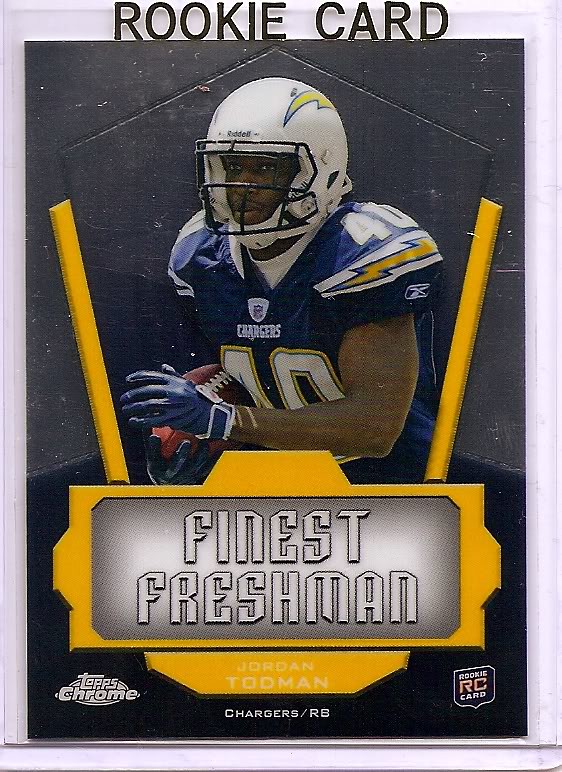This is a detailed image of a Topps Chrome Rookie Card featuring Jordan Todman, a running back for the San Diego Chargers. The card has a white border all around with "Rookie Card" printed in black capital letters at the top. Centered on the card is a photograph of Jordan Todman, an African-American player wearing the Chargers' blue football jersey, which has yellow lightning bolts on the shoulders, and a white helmet with the same lightning design. Todman is carrying the ball in his right arm, with his left arm extended forward, and his jersey number 40 is visible. The player is set against a gray background. Below the photo, there's a yellow box with a silver interior that reads "Finest Freshman" in white text. This box also features two yellow lines extending from the top, resembling goalposts. Directly underneath, it states "Jordan Todman, Chargers R.B." in white text against a yellow strip. The bottom left corner displays the "Topps Chrome" logo, while the bottom right features an emblem.